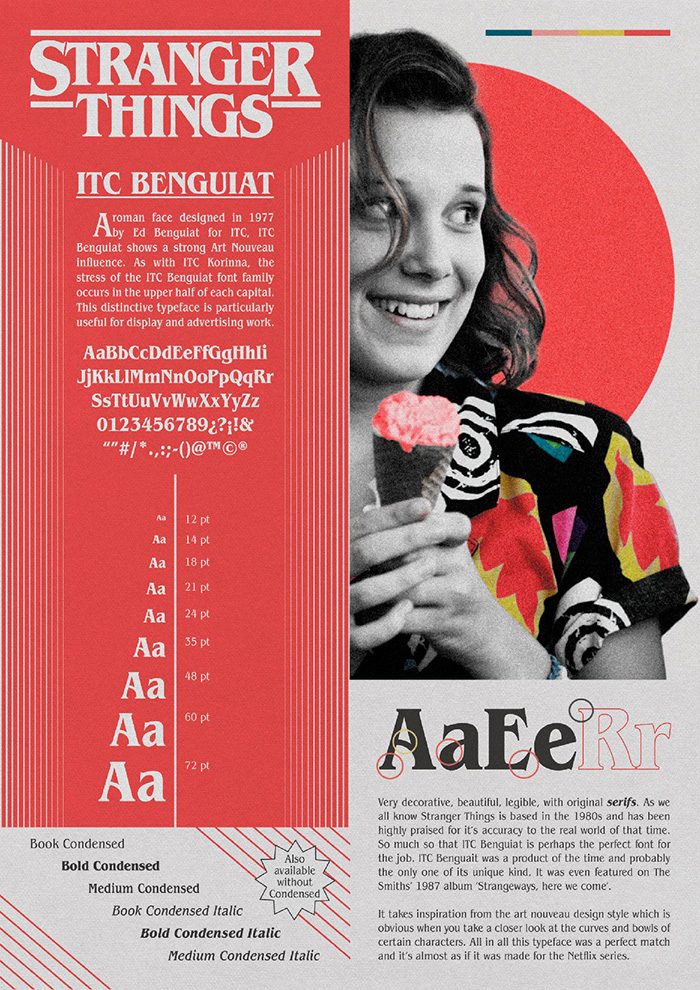In this vintage-inspired Stranger Things advertisement poster, the right side features a teenage girl, Elle, in a predominantly black-and-white image with pops of vivid colors on her shirt, including reds, yellows, teals, and hot pinks. She is smiling and holding a pink ice cream cone with both hands while looking off-camera. The design evokes a nostalgic 1980s vibe, in line with the show's setting. 

To the left, there's a detailed section showcasing the ITC Benguette typeface, described as a Roman face designed in 1977 by Ed Benguette for ITC, renowned for its Art Nouveau influence, particularly evident in the upper-half stress of each capital letter. The typeface is noted for its decorative, beautiful, and legible qualities with original serifs, making it perfect for display and advertising work. This font, featured on the Smiths' 1987 album "Strangeways, Here We Come," is highlighted as an ideal match for Stranger Things, capturing the real-world accuracy of the 1980s. The poster also includes examples of uppercase, lowercase, special characters, and numbers, presented across various sizes and styles, underscoring its versatility and iconic status.